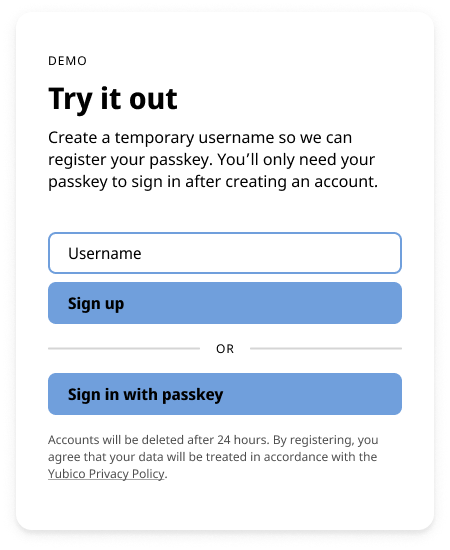The image features a clean, minimalistic interface centered around a white box. At the very top, in unassuming black text, it reads "Demo." Just beneath, in larger, bold black letters, the phrase "Try it out" stands prominently. Below this directive, the text invites users to "Create a temporary username so we can register your passkey. You'll only need your passkey to sign in after creating an account."

Following the instructions, there's a white input field designated for entering a username. Directly underneath this field, there are two interactive blue buttons. The first button, labeled "Sign up," and the second, "Sign in with passkey," both utilize black text for clear readability. 

An additional note clarifies that "Accounts will be deleted after 24 hours," reassuring users about the temporary nature of their trial. It also indicates that "By registering, you agree that your data will be treated in accordance with the Yubico privacy policy," suggesting that Yubico is the company behind this demo platform. The purpose of this interface appears to be encouraging users to experience Yubico's passkey functionality within a limited time frame, albeit without specifying the exact nature of the demo.